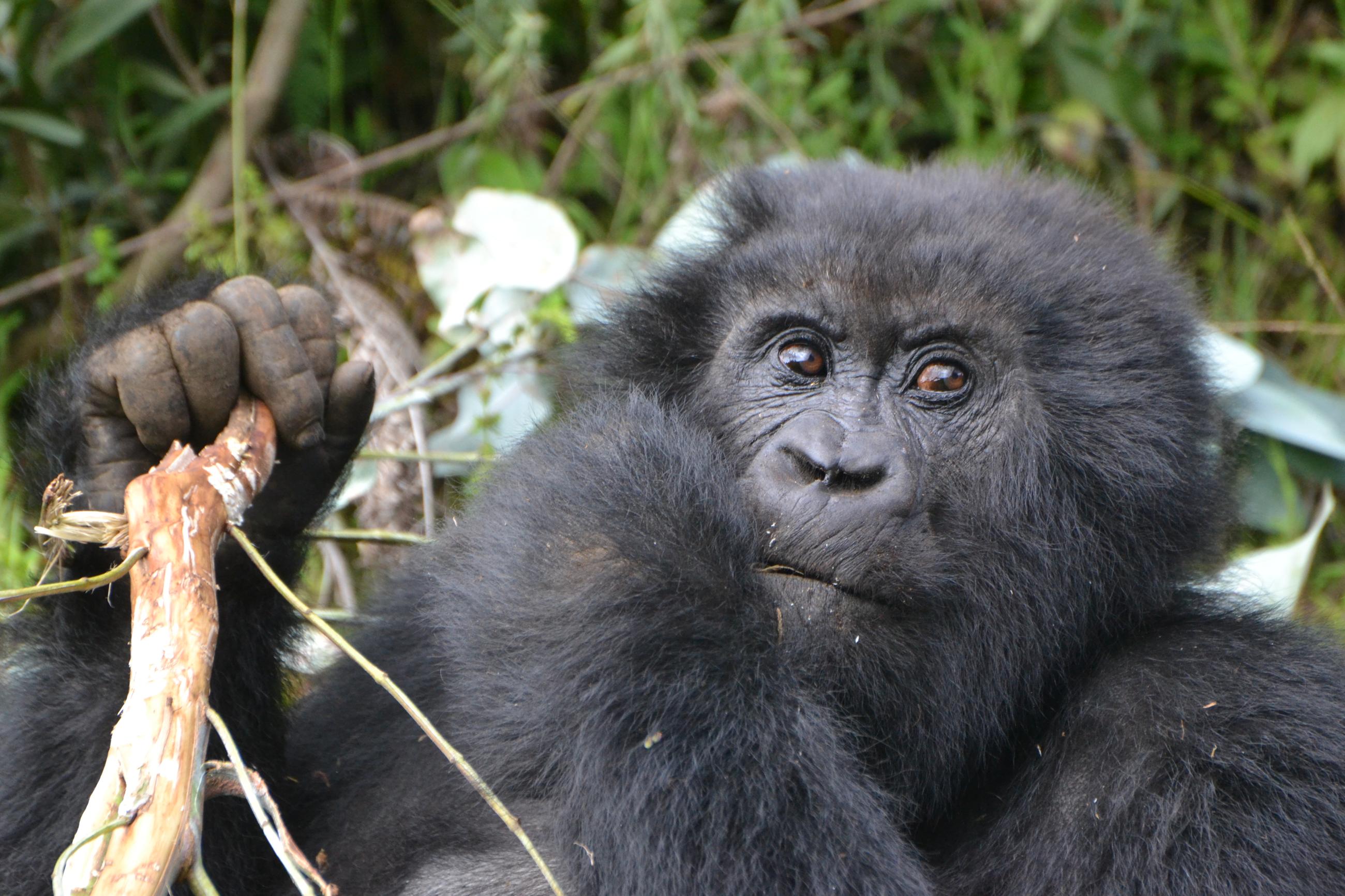This outdoor, rectangular-shaped horizontal photograph captures a close-up of a gorilla in what appears to be a lush jungle setting. The gorilla's black fur appears fuzzy and slightly grayish, and it has expressive brown eyes, although some descriptions hint at a reddish-orange tint. Its face, with a wide, spread-out nose, is prominently featured as it looks slightly to the right. The gorilla is holding onto a large branch with green stems, some of which it seems to be eating. The branch is tan in color, and the gorilla's right hand clasps it firmly. Its left arm is raised, but the hand is not clearly visible. The background features blurred greenery and trees, with some lighter branches and indistinct white patches around the top left and right of the gorilla’s head. Overall, the image beautifully emphasizes the gorilla amid its natural habitat.